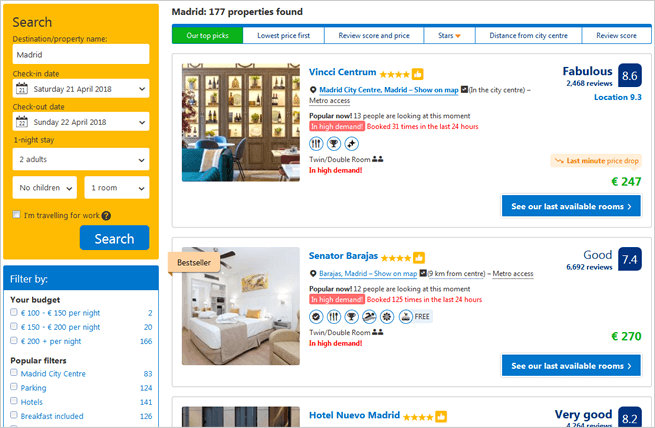The image displays a website interface designed for searching properties, including rental properties, homes, or hotels. In the upper left corner, there is a yellowish-orange search box labeled "Search." This box allows users to enter their desired destination, check-in and check-out dates, the number of people, and the number of rooms required. Below the search fields, there is a search button and an option to check if the user is traveling for work.

Beneath the search box, a filter option is available. To the right, the screen shows a heading that reads "Madrid: 177 properties found." Several tabs are located at the top of the search results, offering sorting options such as "Our Top Picks," "Lowest Price First," "Review Score and Price," "Stars," "Distance from City Center," and "Review Score."

Below these tabs, the search results are displayed, showcasing various property listings with images of the interiors, prices, and user ratings.